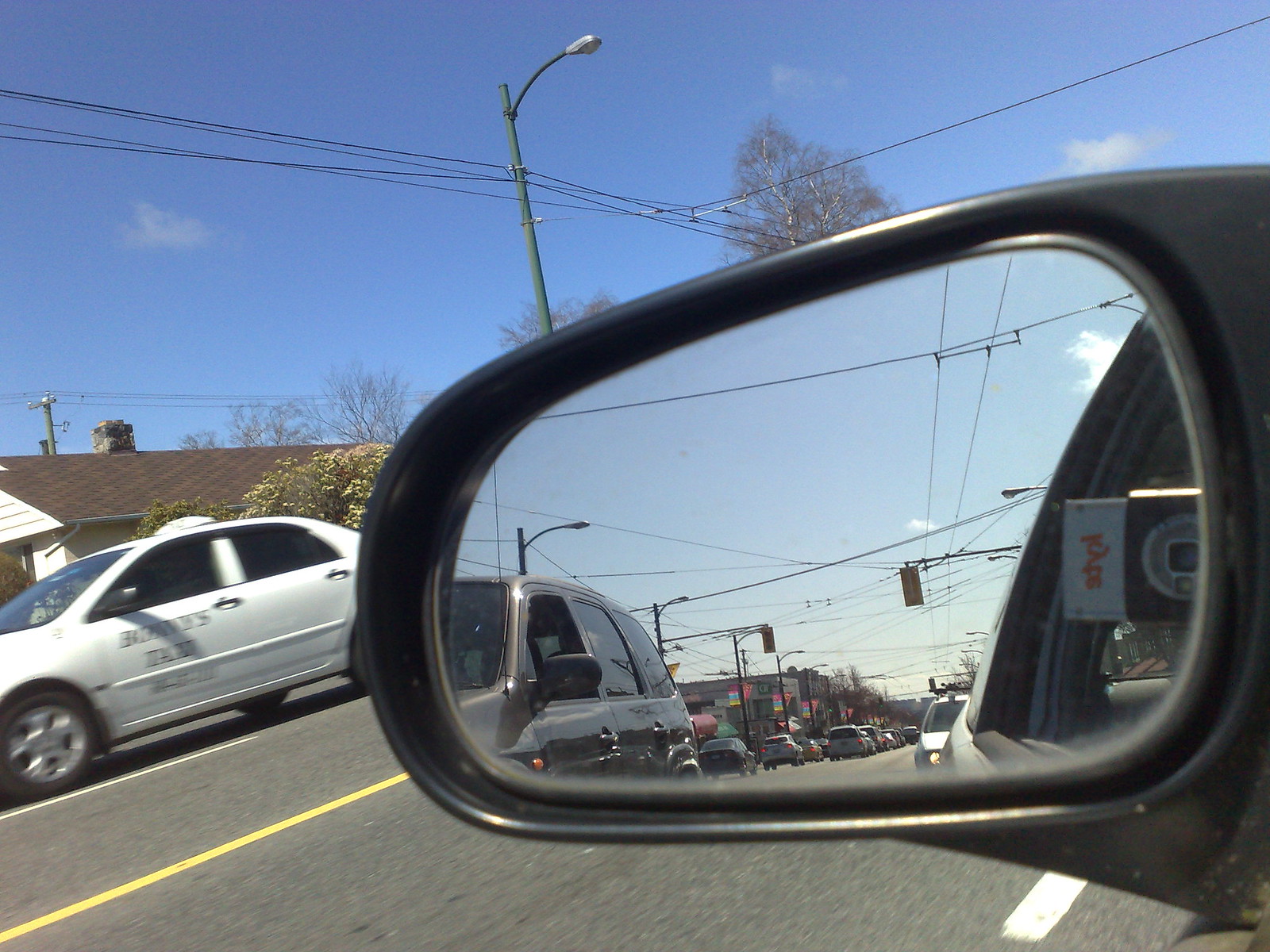The photograph was taken outdoors on a clear, sunny day with a few scattered clouds dotting the azure sky. Overhead, a set of power lines extends from a gray metal pole. In the distance, a tree stands bare with brown, wilted leaves, indicative of the winter season. Dominating the foreground, the side mirror of a vehicle reveals a black SUV approaching from behind. The mirror's black frame also captures reflections of additional power lines, the backs of yellow traffic signal boxes, and a house with a brown roof. A white car, likely a taxi due to the rooftop sign, passes by in the background.